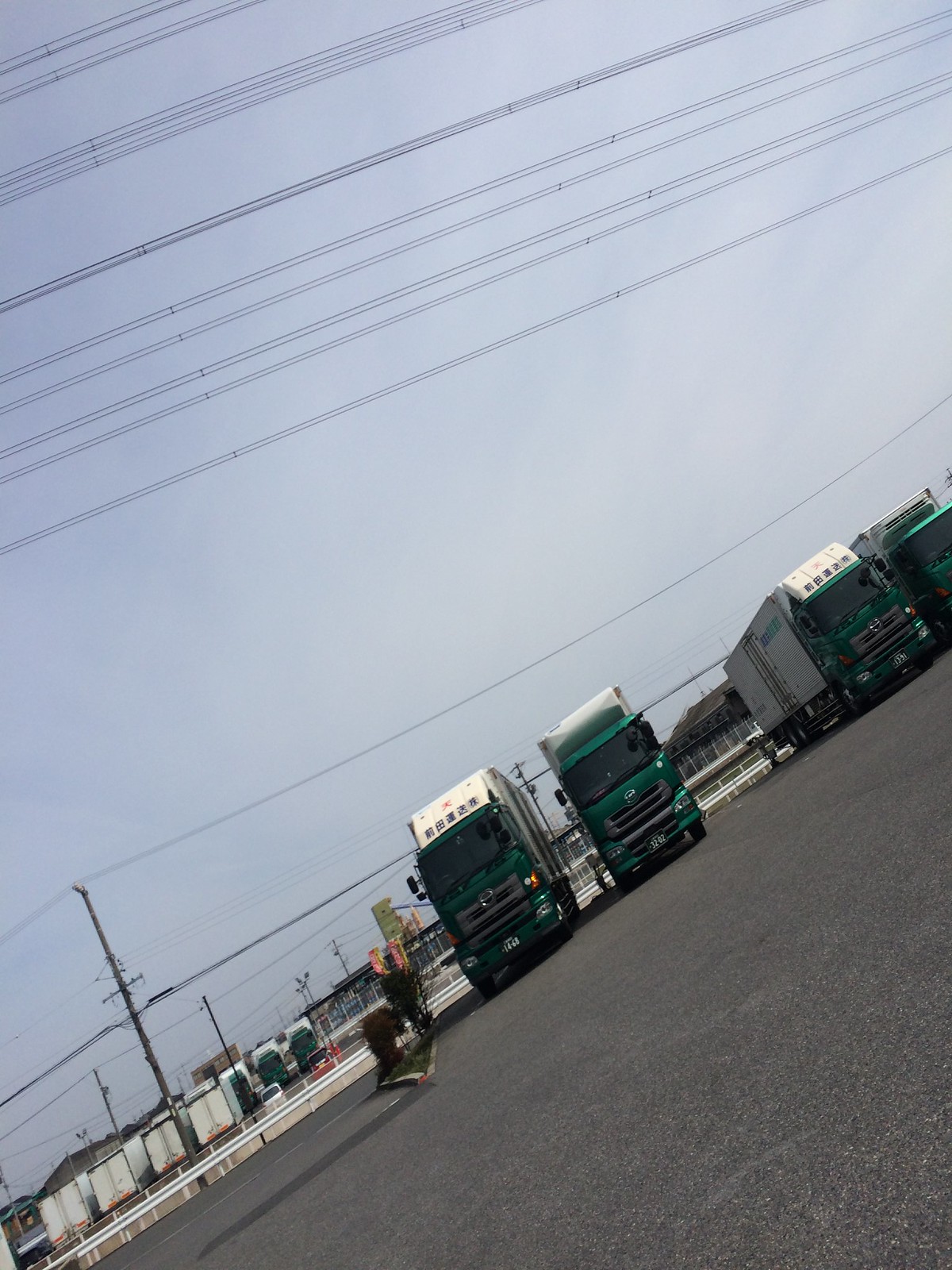The image depicts a slanted scene of a nearly vacant parking lot with a prominent diagonal orientation, making the left side appear lower than the right. Centrally located in the lot are four large, green semi-trucks with black cabs and white trailers. The trucks are distinctively painted with green frames and front parts. Behind these trucks, separated by a rail, is another lot with at least six additional semi-trucks, two of which are the same green color, while the remaining are primarily white from the back view. Above this scene, numerous power lines (approximately 15) crisscross the clear, light blue sky, which appears slightly darker in the top left corner. The photograph is noted for its distorted perspective, potentially taken from a low angle, adding to its unusual, stretched appearance.